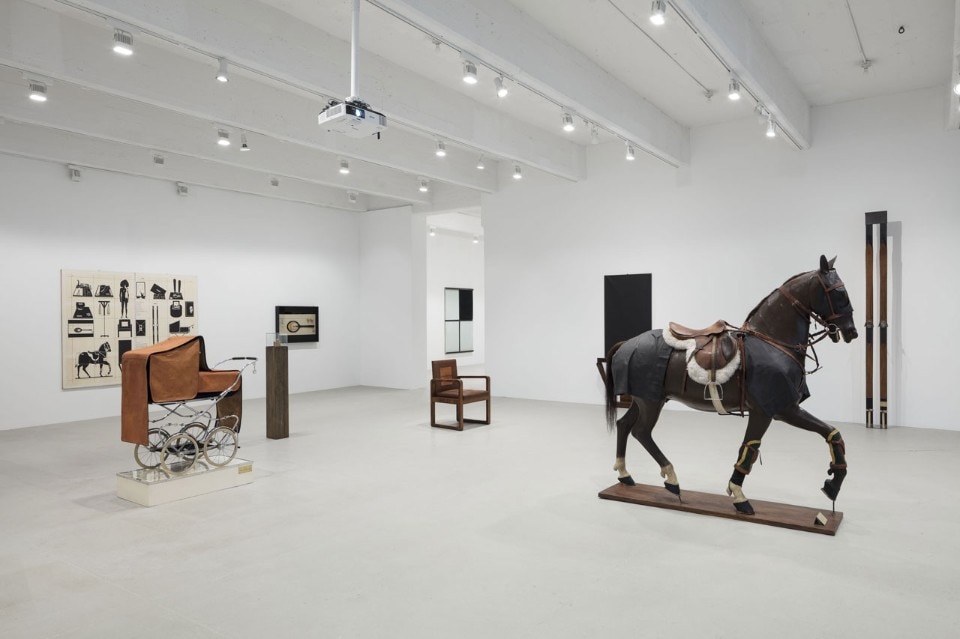The image depicts a sparse, white room, likely an art gallery or museum, illuminated by track and ceiling lights. The floor is light gray-white, complementing the white walls. Central to the scene is a dark, nearly black horse mounted on a wooden stand, with its front left leg slightly raised, as if in mid-prance. The horse is equipped with a bridle, reins, a brown saddle, and a gray blanket draped underneath. Notably, the horse's hooves have white markings and are adorned with cloth just above them.

To the left of the horse stands an old-style baby carriage, or pram, with a black cloth cover and canvas sides. A wooden chair with a brown cushion and square, open-sided wooden frame is also placed in the room. 

The back wall features a painting composed of three white squares and one black square in the upper right corner. Additionally, another artwork depicting horses is visible behind the carriage.

The overall photo orientation is horizontal, capturing the minimalist and serene ambiance of this gallery-like room.